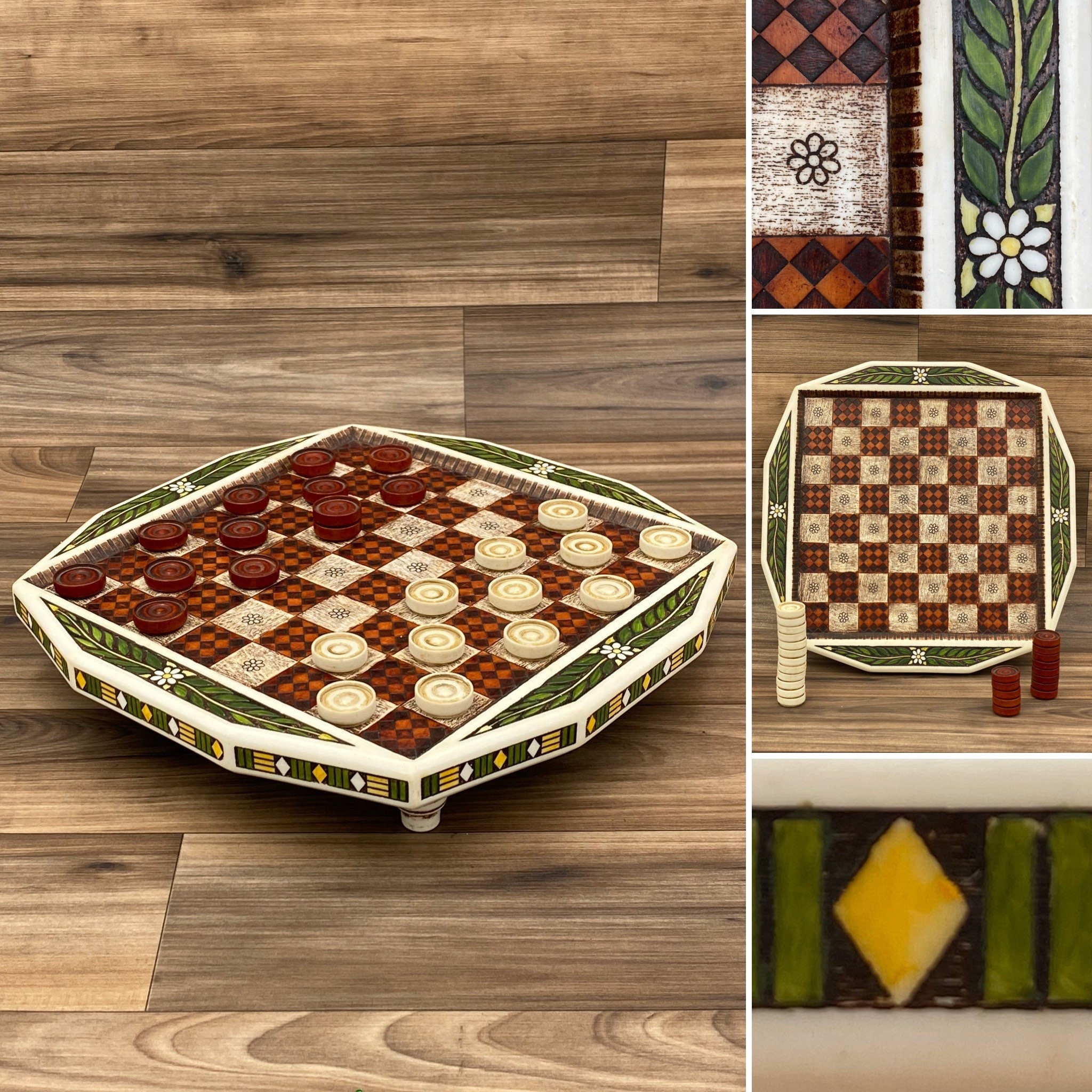This image features a unique and elaborate checkerboard displayed in a composition of four distinct photographs. The largest image, positioned on the left side, showcases the entire checkerboard resting on a wood surface. The board is cream-colored with cream legs and an edge that forms a small lip around all sides. The checkerboard itself is composed of alternating rust-colored squares with orange designs and cream-colored squares with black designs. In the center is a notable white flower with surrounding yellow and white diamond shapes and three green lines.

On the right side, the images are smaller and offer detailed views of the checkerboard. The top-right photo highlights the intricate floral and square designs of the checkerboard with a clear view of the white box and black outlined flower. Below this is another smaller image showing the checkerboard from a side angle, where the top surface and the piles of checkers at both ends are visible. The final image at the bottom-right provides an up-close look at the yellow diamond and the three green lines, offering a detailed glimpse into the board's artistic elements.

Each checker piece on the board features a rust color on one side and a cream color on the other, adorned with a swirl pattern. The board’s artistic and polygonal design, along with its detailed decorative elements, lends it a unique and visually appealing aesthetic.